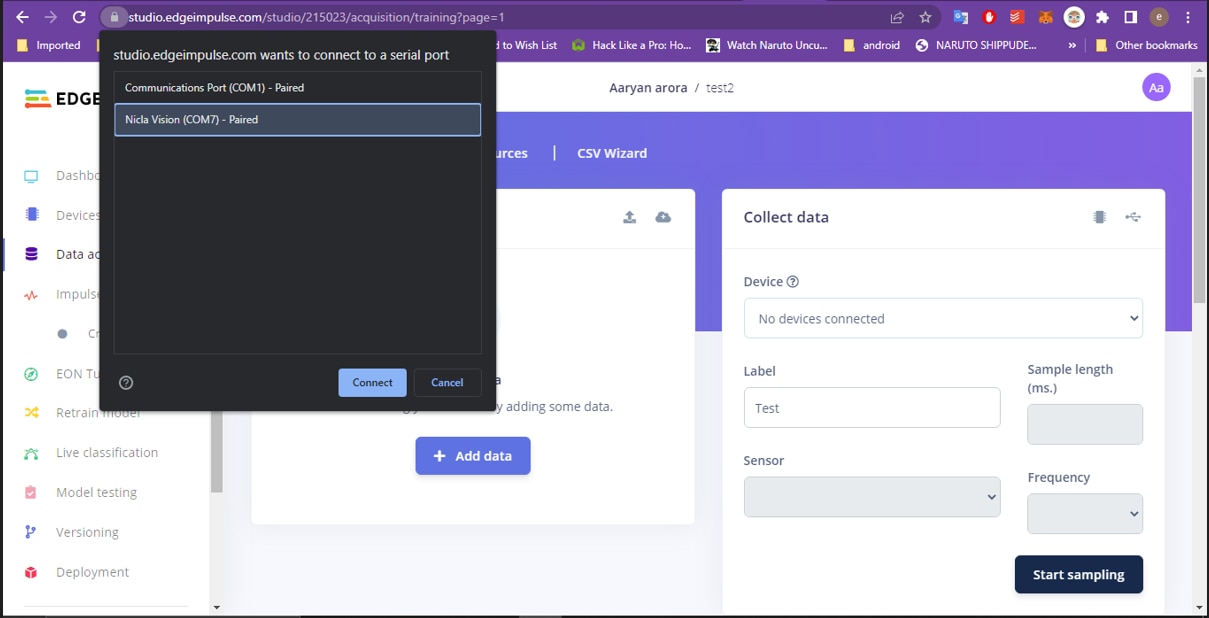The screenshot displays a web browser with a purple-colored browser bar at the top, indicative of a custom or themed user interface. Several shortcut icons are visible on the window, suggesting frequent or easy access to certain functions or websites. The main webpage features a split design: a menu bar on the left, which appears to be dedicated to programming-related functions, and a main content area to the right.

Within the main content area, there are distinct sections. The top section has a white bar, possibly for searching or navigation, followed by multiple purple and white bars containing text. The far-right section is particularly notable, containing a labeled area titled "Collect Data" along with some drop-down menus for user interaction.

Overlaying the webpage is a prominent black pop-up box with the message "studioedgeimpost.com wants access to a serial port." Below the message are two selectable options: the first option, "Communication port COM1 pair," and the second option, which is highlighted in blue, "Niklaavision COM7 (paired)." At the bottom of this pop-up, there are two buttons; a blue "Connect" button on the right and a grayed-out "Cancel" button, indicating the available connection action and the disabled cancel action, respectively.